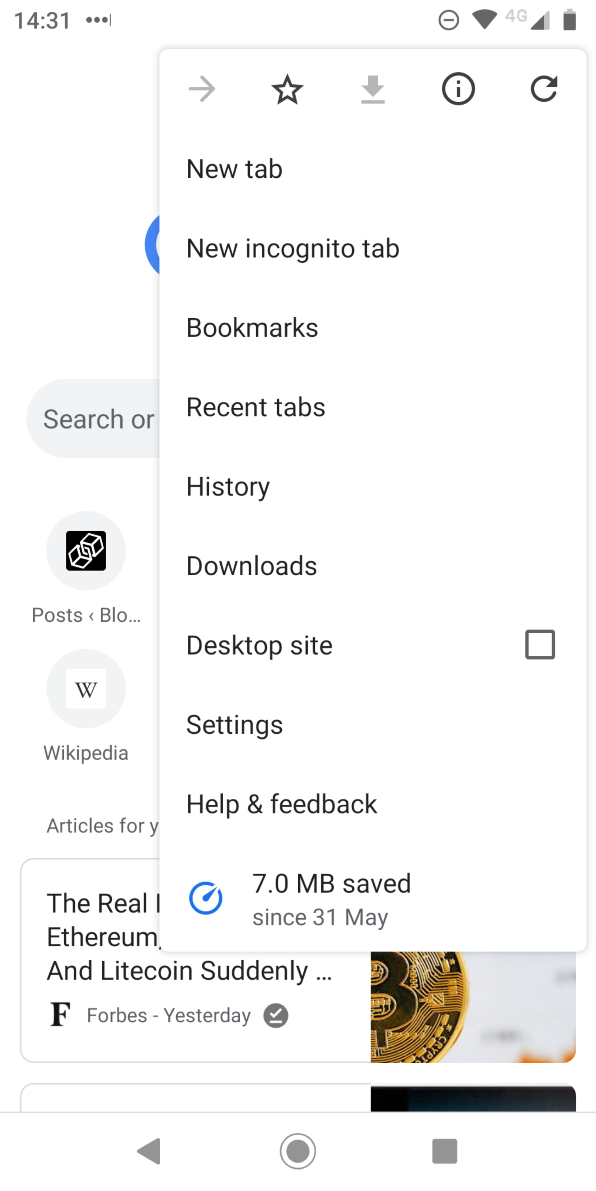The mobile phone screen displays a detailed interface including several icons and informational elements. At the top right corner, indicators show the time as "14:31" or "2:31" along with three dots. A signal icon reveals a strong 4G connection, and the battery icon is full, ensuring prolonged usage. Below these indicators, a box with multiple icons is visible: a right arrow, a star, and a down arrow with a line underneath it, an information 'i' symbol encircled, and a circular refresh arrow.

Just beneath this section, a menu lists various options: "New tab," "New incognito tab," "Bookmarks," "Recent tabs," "History," "Downloads," "Desktop site," "Settings," "Help and feedback," and it notes "7.0 megabytes saved since May 31st." In the background of this box, the Google logo's colors are recognizable, hinting at the Google search page. Partially obscured text says "Search or," and subtitles include "Posts," "Blog," "Wikipedia," and "Articles for you," with a specific article about Bitcoin notably displayed.